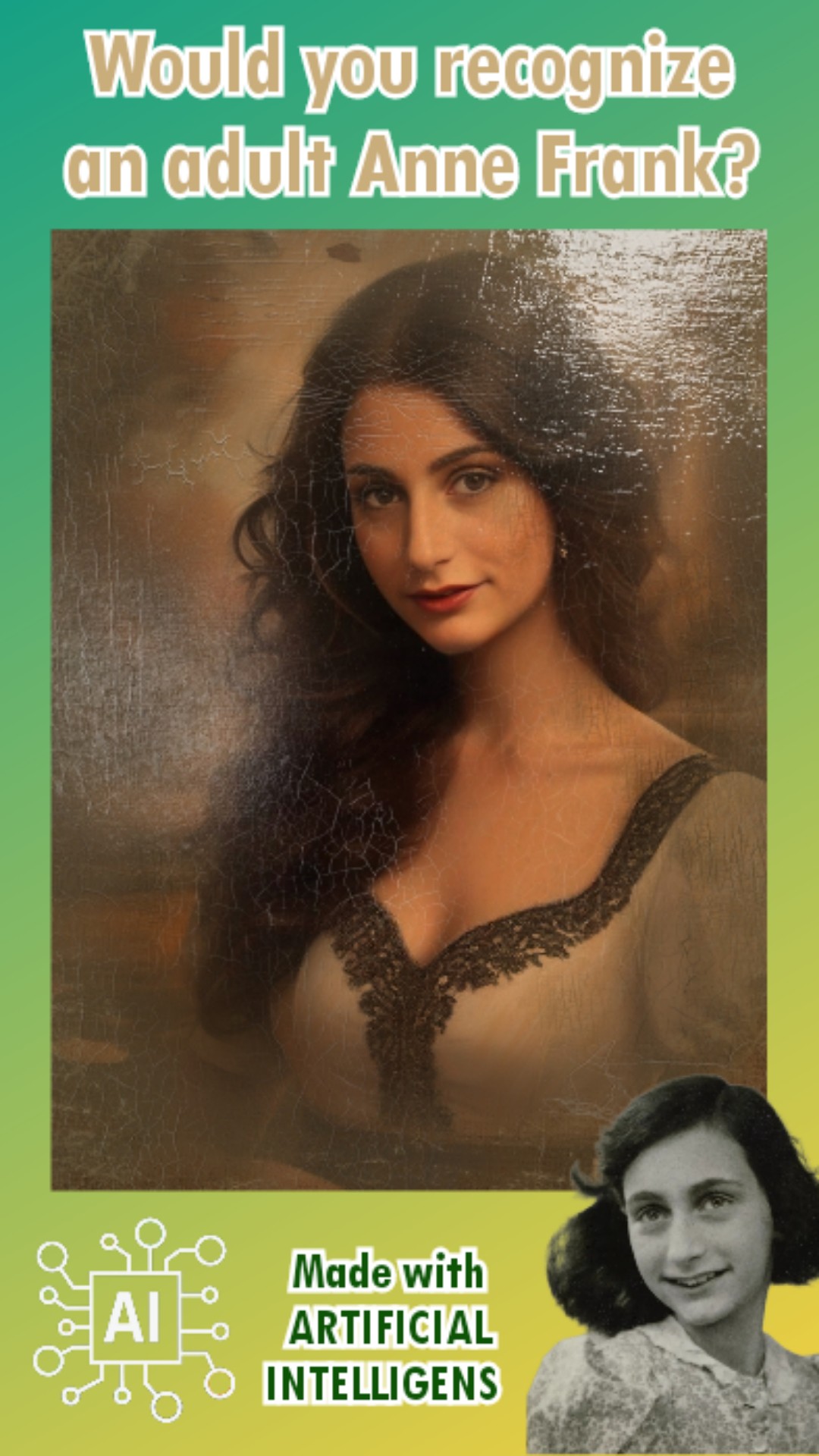The image appears to be an advertisement featuring a simulated depiction of an adult Anne Frank. At the top, in a brownish-gold color, the text poses the question, "Would you recognize an adult Anne Frank?" The central focus is a detailed color portrait of a young woman with long dark hair, dark eyes, and defined dark eyebrows. She is wearing a gray dress accented with black lace around the neckline and bust and has red lips and noticeable makeup. The woman’s serene and enigmatic expression, along with the muted brownish background, invokes a resemblance to the Mona Lisa's iconic style. 

At the bottom right of the image, a smaller black-and-white photo of the real Anne Frank is displayed, accompanied by the text, "Made with artificial intelligence," in green letters. On the bottom left, there's a logo featuring the letters "AI" in a white, boxed square design with lines ending in circles, suggesting a digital or futuristic theme. The overall tone of the image invites viewers to reflect on the capabilities and implications of artificial intelligence, particularly in reimagining historical figures.